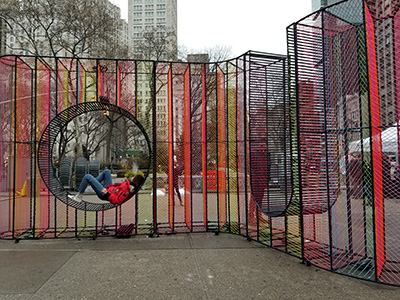In the vibrant city park setting, we see a brightly colored multicolored wire fence, likely between 8 and 10 feet tall, that forms an enclosure resembling a playground area. At the center of this fence, there is a large black wheel, similar to a hamster wheel, suspended for people to interact with. Reclining inside this wheel is a woman dressed in blue jeans and a red jacket, her brown hair cascading over the upper part of the wheel. The area surrounding them consists of gray asphalt walkways where several other people are walking. The scene is adorned with tall and short trees, hinting at an autumn setting as they prepare to shed leaves. In the distance, there's a white tent positioned on the hard court of the playground, and several towering buildings, including a prominently tall white building, and a 20-story apartment complex, all under a mostly cloudy, white sky typical of a daytime scene.